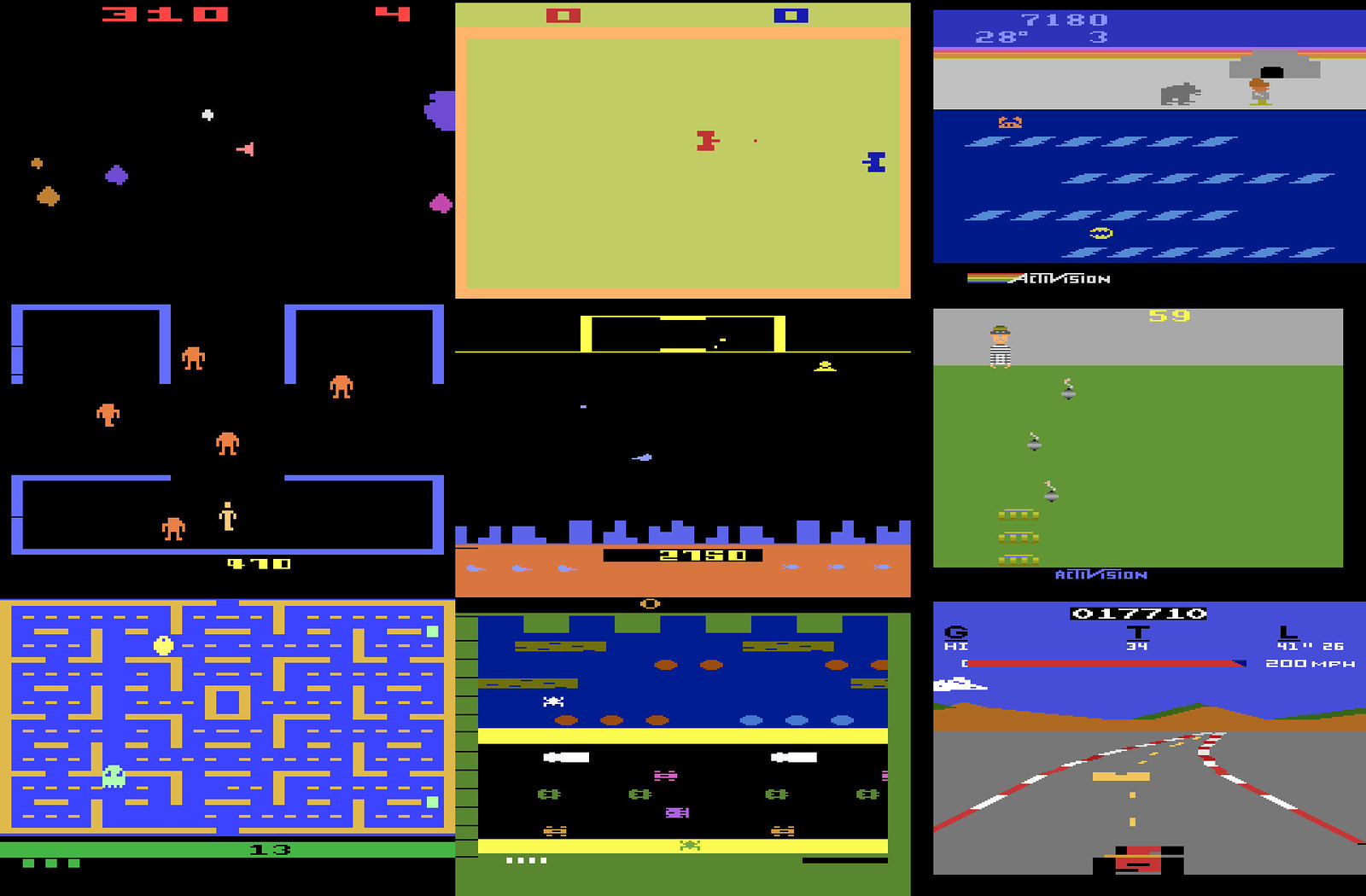The image showcases a grid of nine screenshots from vintage 8-bit Atari video games, arranged in a three-by-three pattern. The top row features, from left to right, Space Invaders, Joust, and an unidentified game with an elephant-like figure. The middle row includes Donkey Kong on the left, a variant of Space Invaders in the center, and what appears to be Ridge Racers on the right. Finally, the bottom row displays Pac-Man on the far left, another variant of Space Invaders in the middle, and a racing game on the lower right corner. Each screenshot presents pixelated graphics iconic of classic arcade games, depicting a variety of activities ranging from interstellar battles and racing to polar adventures and classic arcade competitions.